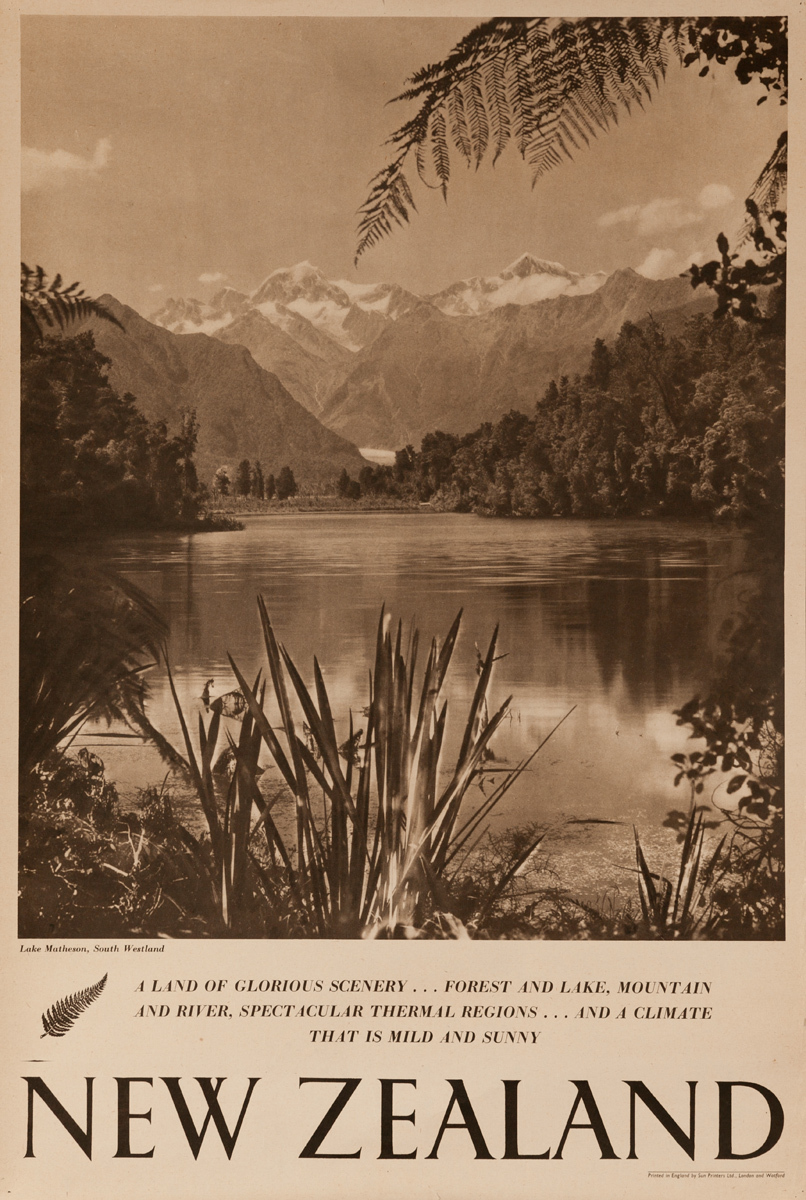This aged black-and-white or sepia-toned poster, likely a vintage magazine advertisement, showcases the breathtaking allure of New Zealand. Dominating the poster is a large, clear image of Lake Matheson in South Westland. The lake is bordered by an array of trees, bushes, and fronds, with some larger leaves overhanging the serene water. In the background, majestic snow-capped mountains rise against a sky dotted with clouds. Detailing the natural beauty of the region, text at the bottom in large bold lettering simply states "New Zealand." Above this, smaller text describes the country as "a land of glorious scenery... forest and lake, mountain and river, spectacular thermal regions... and a climate that is mild and sunny." The overall sepia tone and old-fashioned font suggest the poster dates back to an earlier era, enhancing its nostalgic charm.